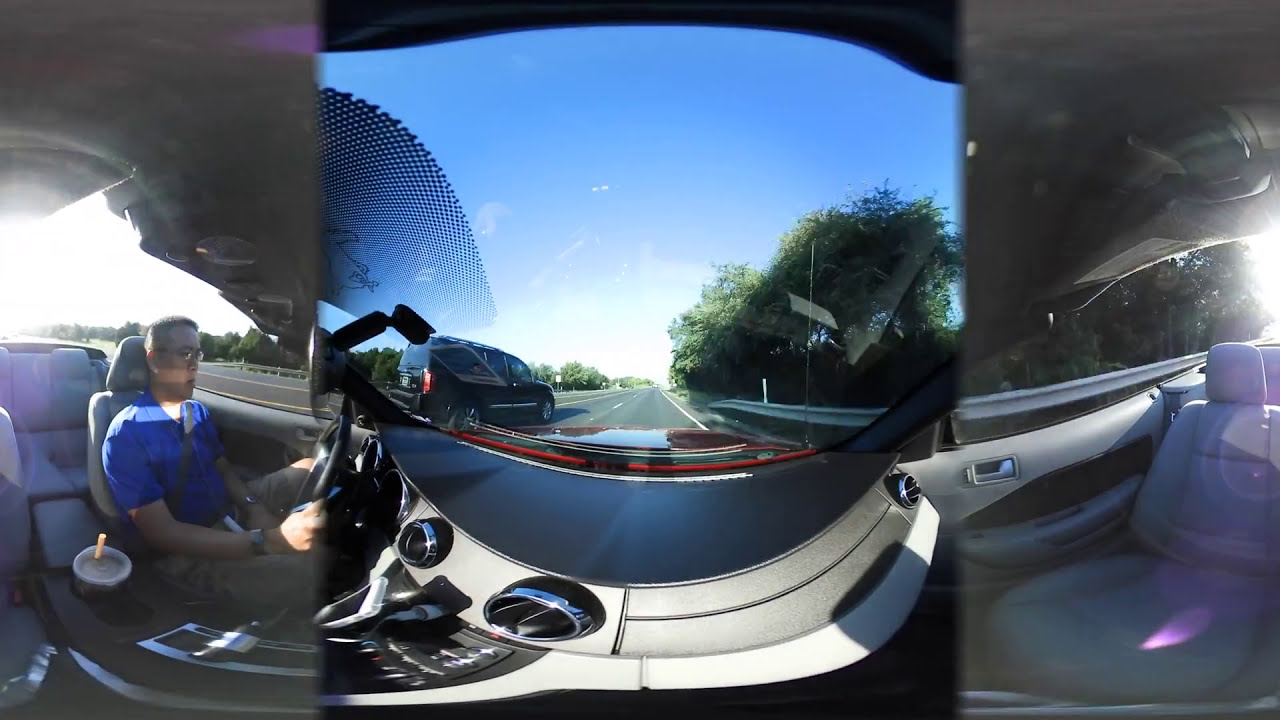The image is a horizontally-aligned rectangular shot, captured inside a convertible car using a 360-degree wide-angle lens, resulting in a slightly distorted view. Central to the image is a clean and clear windshield, through which you can see a sunny sky with a few white clouds towards the horizon. The car is driving down a two-lane road, with a dashed white line separating the lanes and a solid white line on the right, next to a guardrail. To the left, there's a black SUV in the adjacent lane. Large trees line the right side of the highway.

On the left side of the image is the driver, appearing to be an Asian man with short dark hair, wearing glasses and a blue short-sleeve polo shirt. His right hand is on the steering wheel, and there's a drink in the cup holder next to him. The seats, which are gray leather, suggest a high-end interior. The dashboard stretches and curves due to the wide-angle perspective. The passenger seat next to the driver is empty, and parts of the console and door panel on the passenger side are slightly blurred. The sun shines brightly, casting a clear light inside the car. The driver’s face shows no visible emotion, as he focuses on the road ahead.